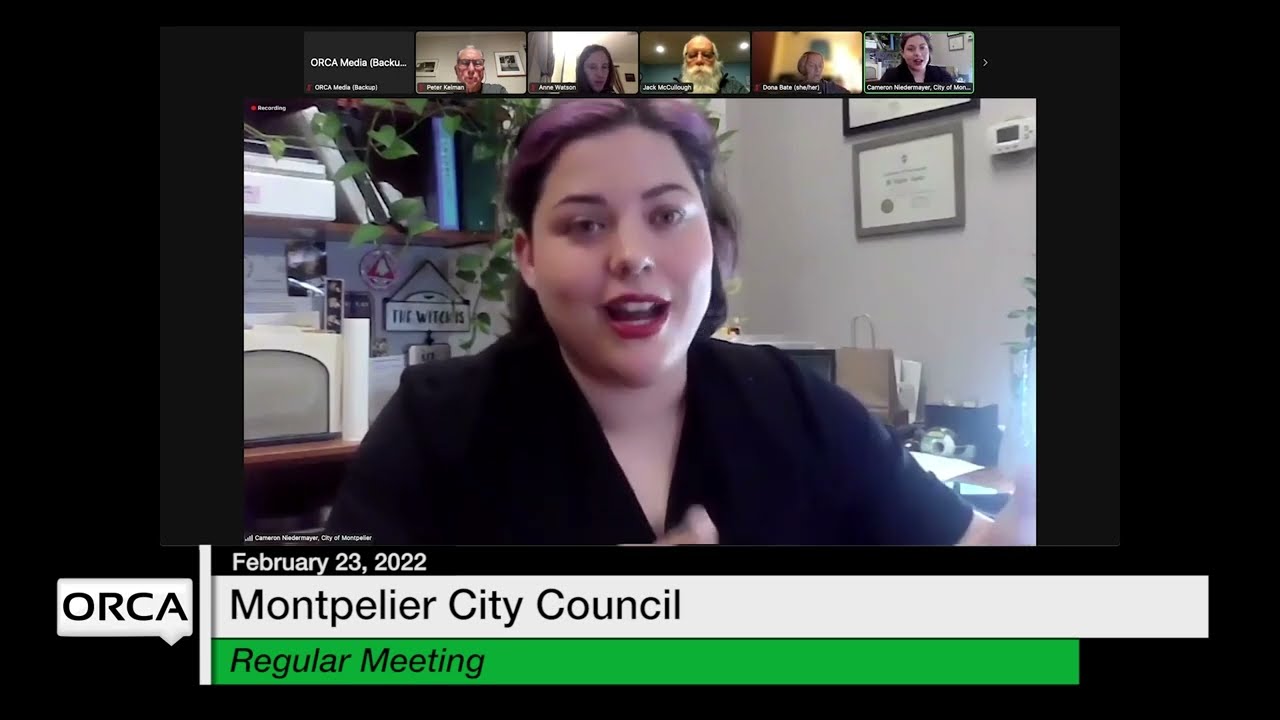This image depicts a screenshot from a Zoom meeting of the Montpelier City Council, conducted on February 23rd, 2022. The foreground showcases a woman mid-speech, her webcam image prominently featured. She is wearing a short-sleeved black shirt, red lipstick, and has purple-dyed hair with either a headband or glasses perched on top of her head. The setting behind her is an office environment, complete with office supplies, binders, certificates, and a roll of tape on her desk. Above her, a thumbnail panel displays images of other meeting participants, with their names listed. The screen header indicates "Orca Media" and below it, "Montpelier City Council, Regular Meeting" with the text “Regular Meeting” clearly marked, with "Regular" in a green rectangle. The screenshot captures the collaborative nature of this virtual council assembly.